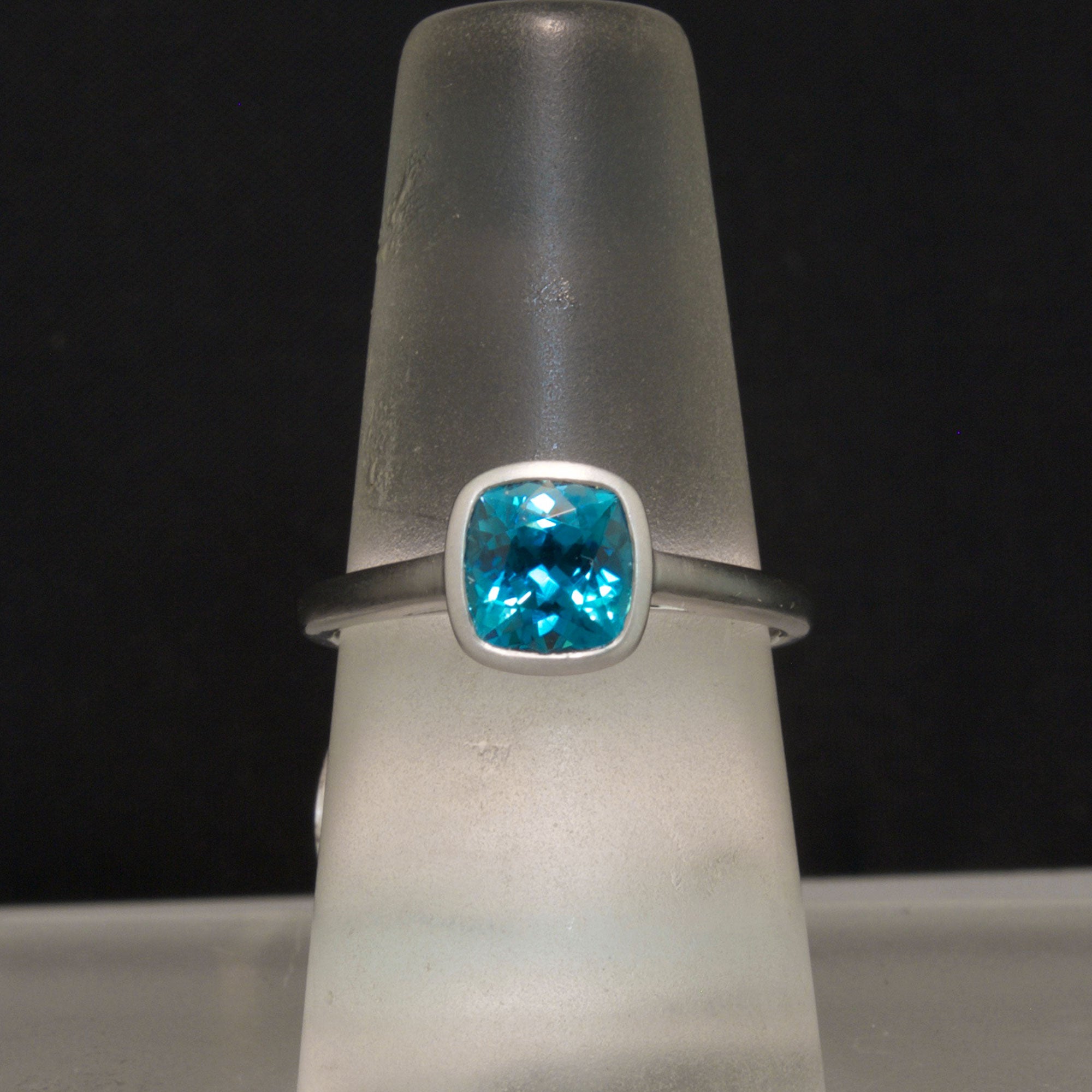The image shows a detailed view of a silver metal ring placed on a semi-transparent, jelly-like, white cone-shaped stand, which is likely used for measuring ring size. The background is stark black with a gray platform at the bottom. At the center of the ring is a square-shaped, faceted blue gemstone that shines with white reflections. The gemstone is held securely within a silver metal setting, adding a touch of elegance to the overall composition. The contrast between the black and gray background and the vibrant blue stone draws attention to the intricate details of the ring and its setting.